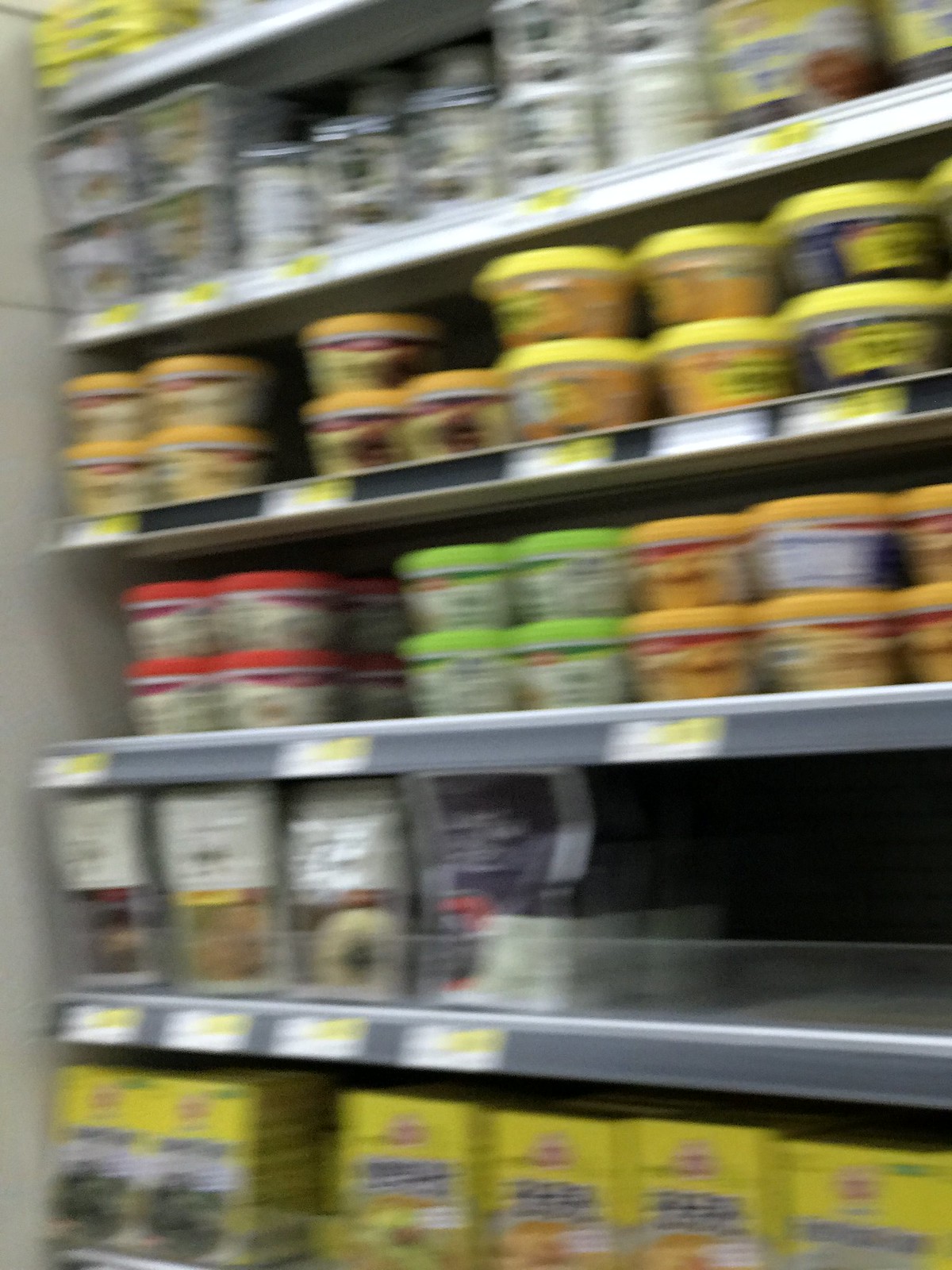A blurred image of a supermarket aisle, distinctly foreign in appearance, reveals six visible shelves stocked with various products. The bottom shelf is lined with uniformly branded yellow boxes, differentiated by assorted color markings and adorned with a distinct red logo, indicative of different varieties within the same product line. Above it, packets of an unidentified product occupy the next shelf. The subsequent four shelves are neatly arranged with single-serve microwavable containers, consistently branded with variations in flavor or type, further enhancing the diverse assortment available in this unfamiliar supermarket setting.